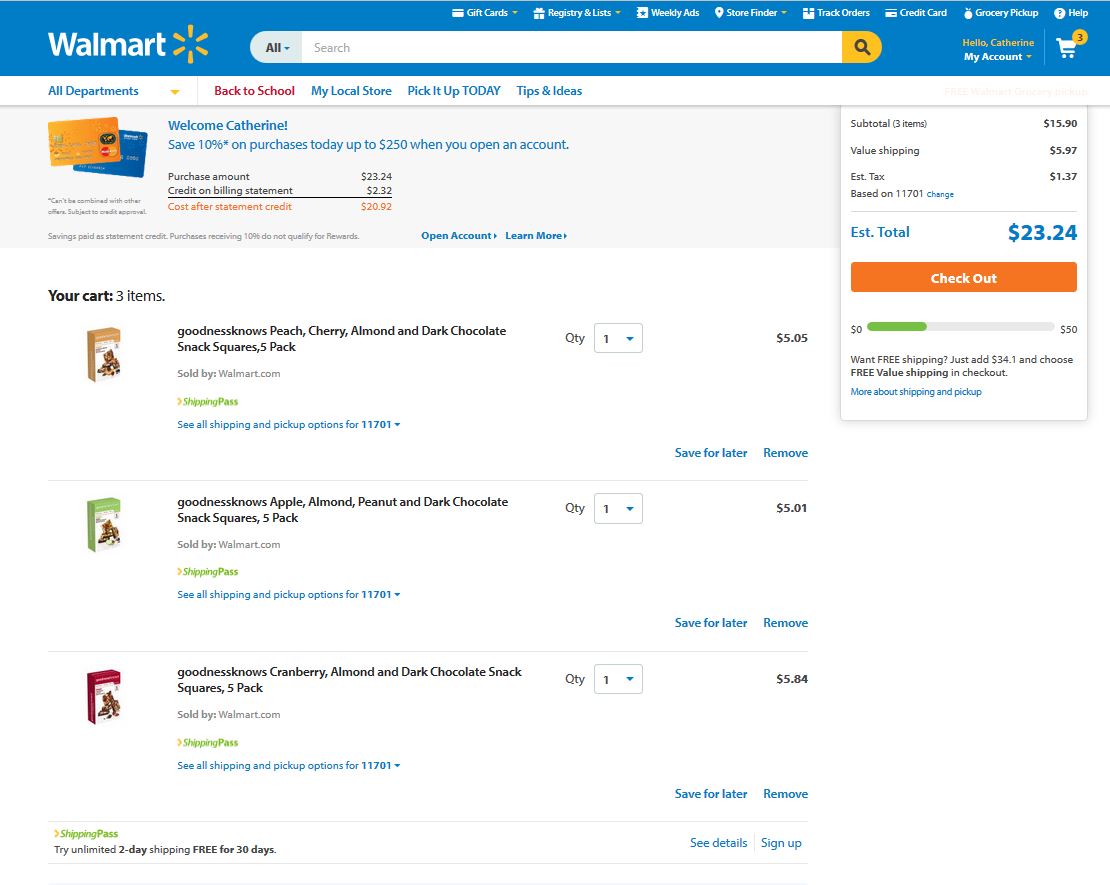A detailed page from Walmart's website is displayed, showcasing various elements geared towards user convenience and personalization. In the upper left-hand corner, the Walmart logo featuring their yellow flower insignia is prominently visible. Adjacent to it, a top navigation bar provides access to various categories, including "Gift Cards," "Registry," "Ads & Weekly Ads," "Finder & Track Orders," "Gift Credit Card," "Grocery Pickup," and "Help."

In the upper right corner, there is a shopping cart icon with an orange circle showing the number "3" in black, indicating the items in the cart. Next to it, a personalized greeting reads, "Hello, Catherine," followed by options like "My Account," making the user experience more personalized.

Beneath the header is a white bar, predominantly blue except for the search bar, with white lettered links to sections like "All Departments," "Back to School" (highlighted in red), "My Local Store," "Picked Up Today," and "Tips and Ideas." An advertisement on the bar extends a personalized welcome to Catherine, offering a 10% discount on purchases up to $250 when she opens an account.

On the right side of the page, details of Catherine's shopping cart are outlined: her subtotal is $15.90, value shipping costs are listed, and an estimated tax amount is included, bringing the estimated total to $23.24, highlighted in blue. An orange "Checkout" button with white text stands out, accompanied by a progress bar below it showing how close Catherine is to completing her purchase; the bar is slightly green on the left and predominantly white.

Inside her cart, detailed subtotals show she has three items. Each item is characterized by categories and flavors, with all of them being snacks but in varying flavors. Additionally, positive messages such as "Good news" may be displayed, emphasizing the beneficial aspects of her shopping choices. 

This entire web page layout emphasizes ease of navigation, personalized service, and clarity of information for the user.